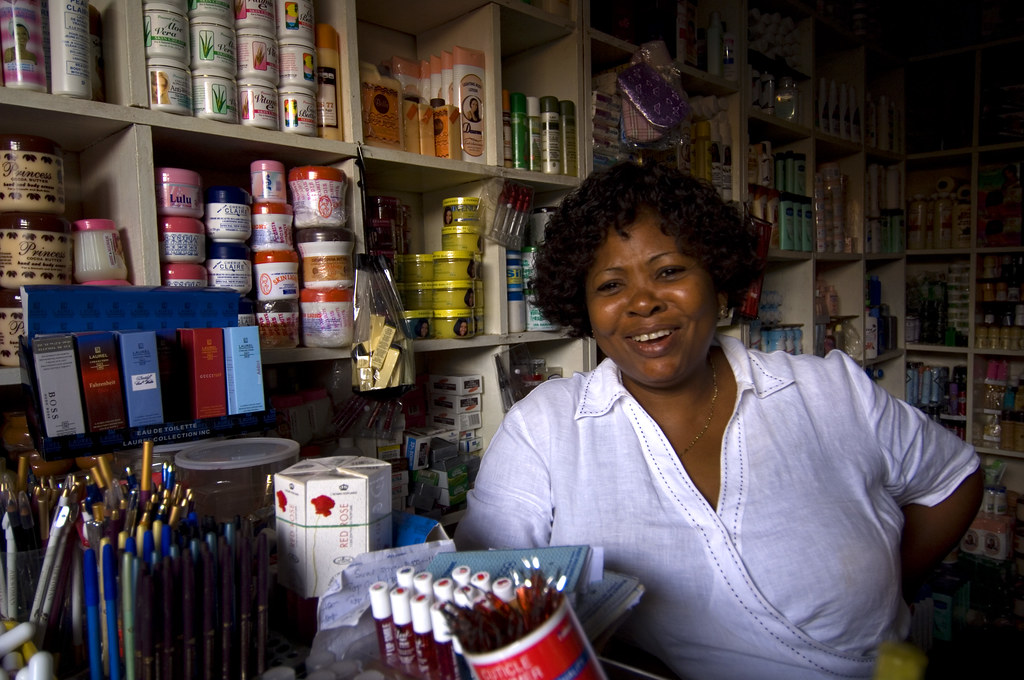In the image, a large African-American woman with dark skin and short, curly black hair stands smiling and looking directly at the camera, exuding happiness. She is adorned in a light blue outfit with a white collar, possibly resembling a maid’s uniform, and wears a very small necklace. Her left arm is confidently placed on her hip. To her right, there is a display of boxed colognes and containers, some likely used for cuticles, along with jars filled with pencils and pens. These items are arranged prominently on the counter in front of her, giving the impression she might be running the store. Behind her, the background reveals walls lined with cube shelves, each filled with various products including shampoos, hair gels, nail health items, and possibly some cleaning supplies. The shelves and products fade into darkness towards the back, creating a strong sense of depth in the store's layout.